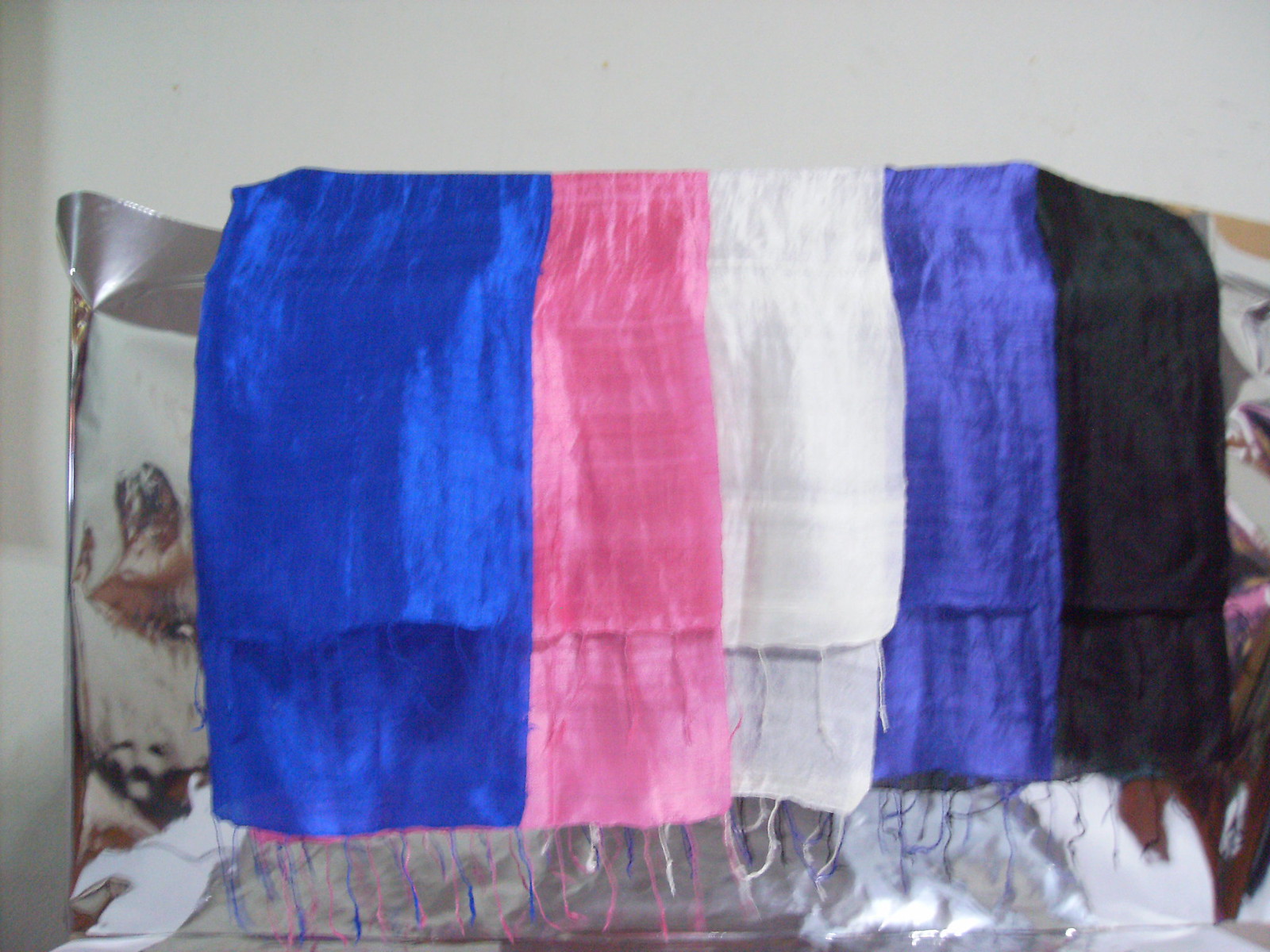The image depicts an indoor setting with a grayish or off-white wall that runs from the upper left to the upper right and down the left side of the photo. Draped over a pillow, adorned with a dog print in tan, green, gray, and silver hues, are five scarves or shawls. The scarves are arrayed in a sequence from left to right: a blue one with blue tassels, a pink one with pink tassels, a white one with white tassels, another deeper blue one that might appear purplish due to light reflection, and a black one with black tassels. Each of these scarves features pointed, fringed ends. Beneath the scarves at the bottom of the image, there's an additional piece of gray fabric. The scarves are laid out in such a way that it's unclear whether they are individual pieces or part of a longer, interconnected piece.